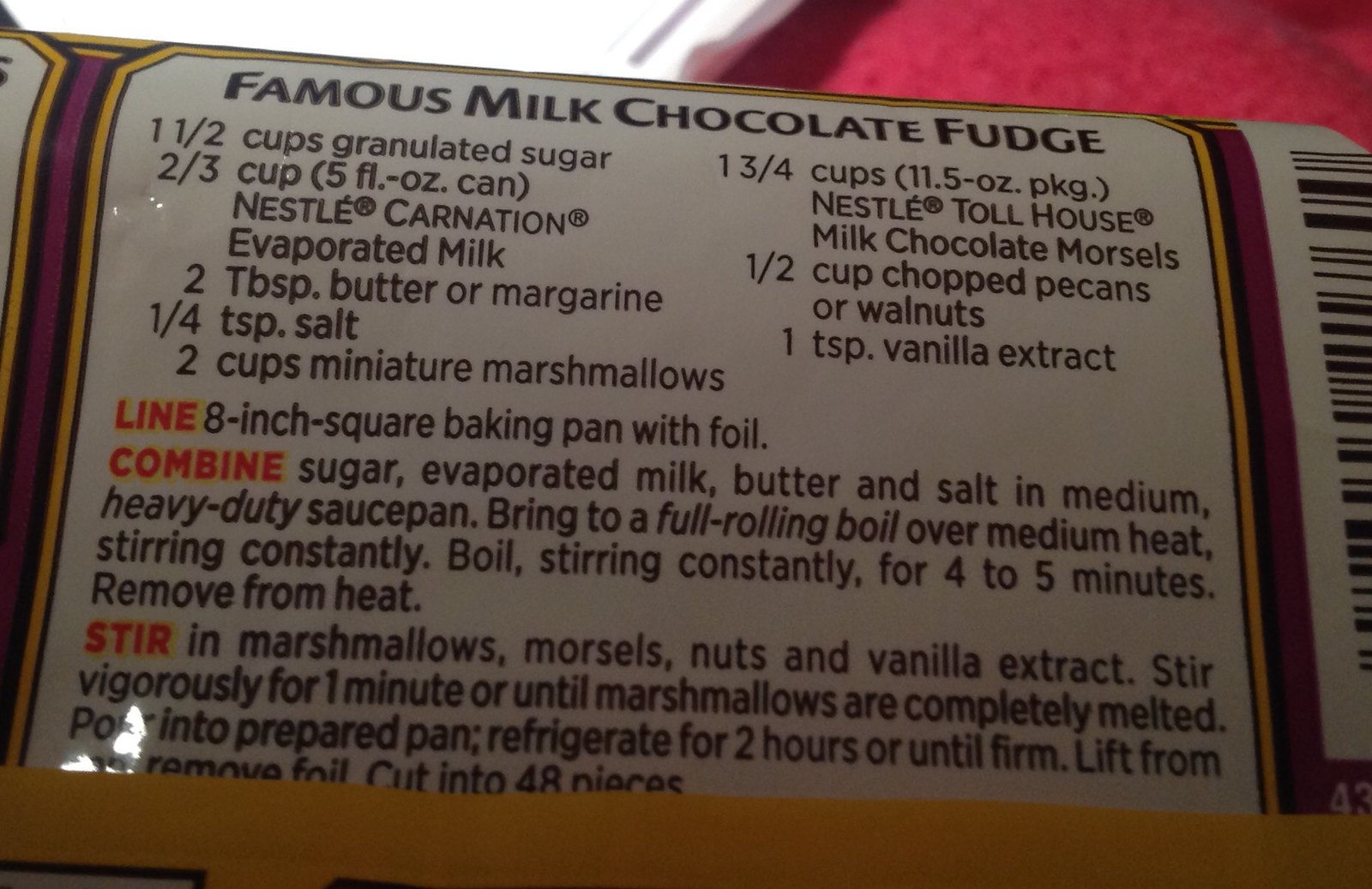This detailed close-up photograph features the back of a plastic Toll House chocolate chip package, specifically zoomed in on a recipe for "Famous Milk Chocolate Fudge." The recipe is displayed within a rectangular yellow and black border, with accents of purple on the sides. The image also shows a pinkish area in the top left corner, while the rest of the background is white.

The recipe itself lists the ingredients: one and a half cups of granulated sugar, two-thirds of a cup or five fluid ounces of Nestle Carnation evaporated milk, two tablespoons of butter or margarine, a quarter teaspoon of salt, two cups of miniature marshmallows, one and three-quarters cups or an 11.5 ounce package of Nestle Toll House milk chocolate morsels, half a cup of chopped pecans or walnuts, and one teaspoon of vanilla extract. 

Instructions are written with certain key steps emphasized in red letters. It reads: "Line an 8-inch square baking pan with foil. Combine sugar, evaporated milk, butter, and salt in a medium heavy-duty saucepan. Bring to a full rolling boil over medium heat, stirring constantly. Boil, stirring constantly for four to five minutes, then remove from heat. Stir in the marshmallows, morsels, nuts, and vanilla extract. Stir vigorously for one minute or until marshmallows are completely melted. Pour into the prepared pan. Refrigerate for two hours or until firm. Lift from and remove foil, then cut into 48 pieces."